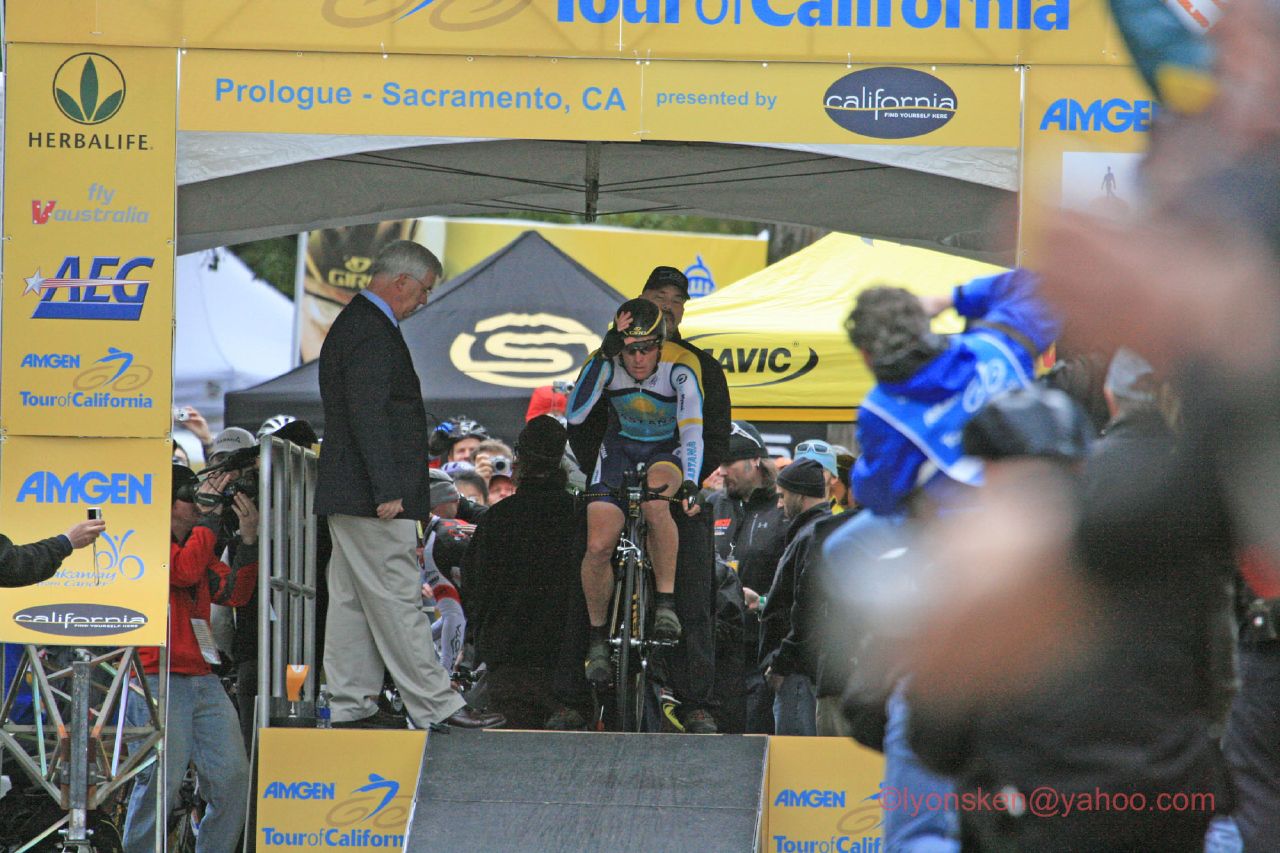This detailed outdoor photograph captures a cyclist crossing the finish line during a race event, likely set in California, as suggested by several sponsorships displayed prominently on a large yellow archway labeled "Prologue Sacramento, California" and featuring logos such as Amgen, Herbalife, and Tour California. The man on the bike is clad in white, yellow, and blue biking gear, with a black helmet and black shoes, poised to descend a black ramp towards the finish. A notable feature is a man in khaki pants and a navy blue blazer to the left, attentively watching the cyclist, while another man in blue is seen photographing the moment from the back. The scene is bustling with a crowd of spectators and photographers, all keenly capturing the race conclusion. The photograph, basking in daylight, exudes a sense of excitement and achievement as onlookers clap and cheer amid a backdrop of sunny weather. The image is distinctly marked with copyright text in the bottom right corner, reading "lyonsken at yahoo.com".